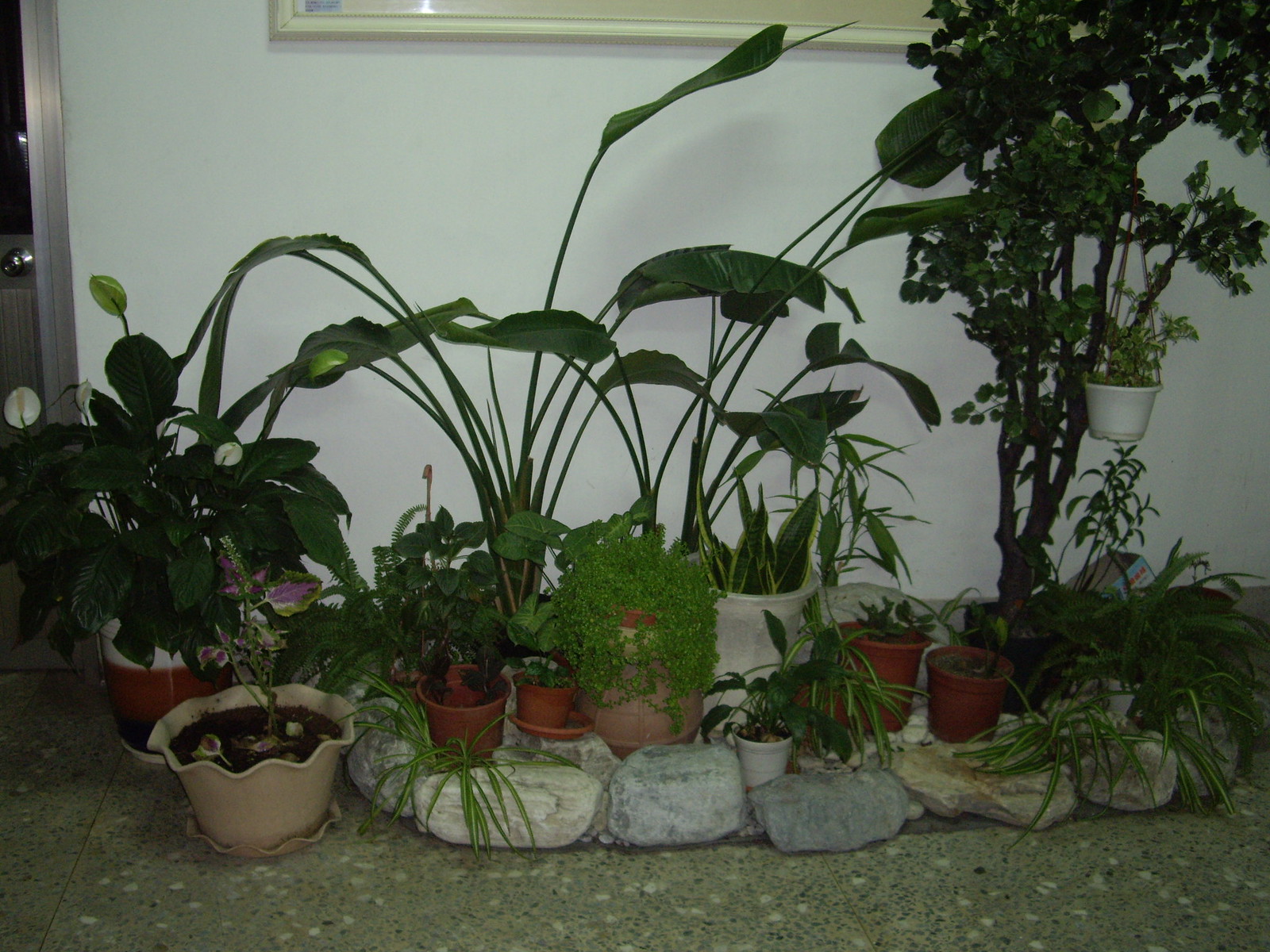The image features a variety of potted plants, meticulously arranged against a white wall. The plants are diverse in type and size, ranging from tall and skinny to short and shrubby, with hues varying from light to dark green. Notably, towards the left, a plant in a light brown pot has distinctive pink and green leaves. The pots, which include terracotta and white ones, are set atop an oval cement stone structure that is slightly elevated above a speckled gray tile floor. A white picture frame and the metal frame of a door with its handle are visible in the upper corners of the image. The photograph appears to have been taken at night, using flash to illuminate the scene.